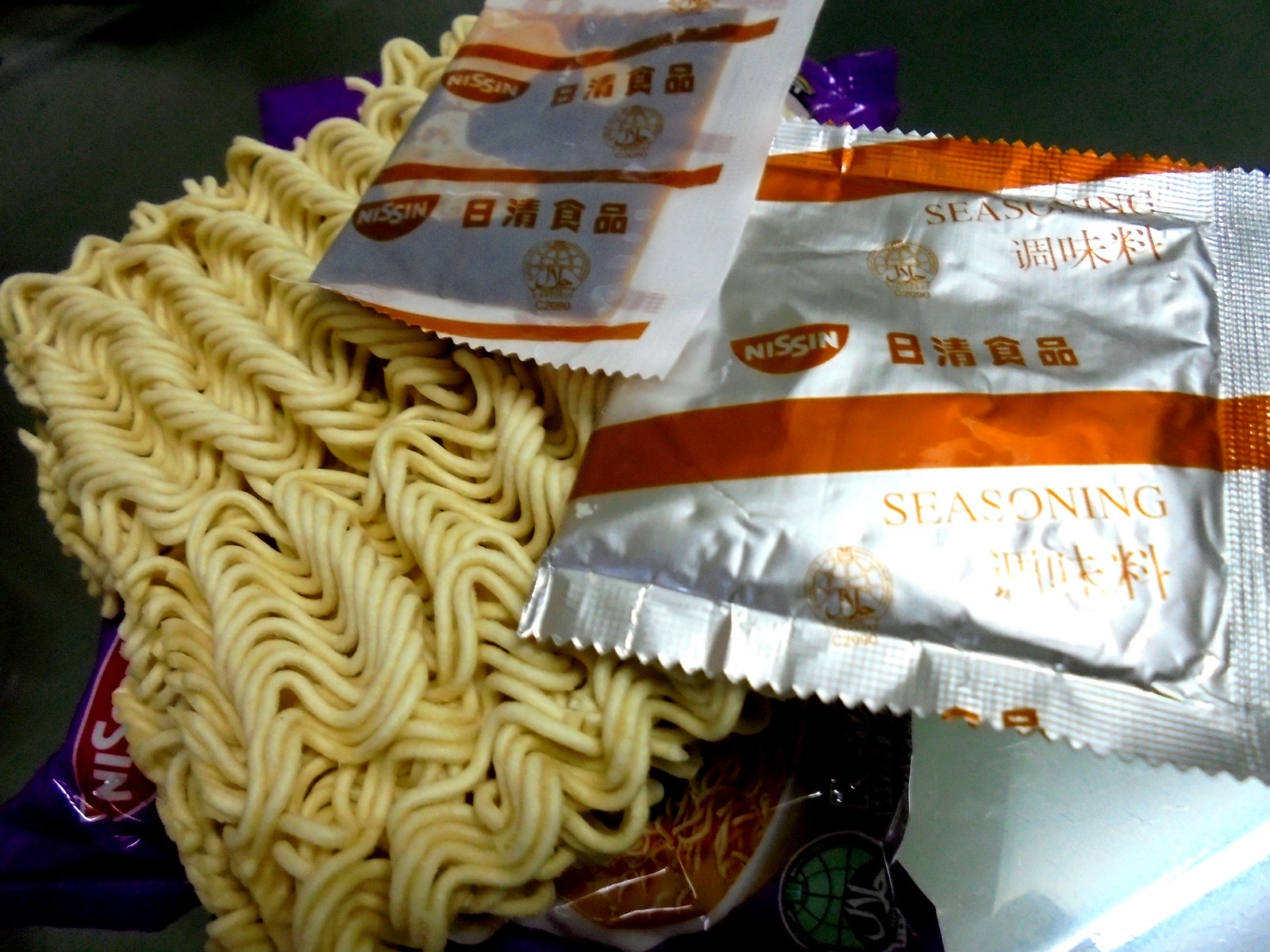The image showcases a close-up view of dry, swirly ramen noodles, prominently placed on the left side against a red plastic backdrop. Two silver seasoning packets are positioned on top of the noodles. Each packet features distinct orange stripes and a semicircle with the text "NISSIN" in its center, surrounded by Japanese characters. The packet closest to the upper right corner has a bold orange stripe and the word "seasoning" prominently displayed, with a notable reflection adding a bright highlight. There's also an orange half-moon symbol near the center, bordering more foreign text. Further details include a diagonal blue streak with a light blue shadow on the bottom right corner and solid black on the other corners. Behind the noodles and packets lies a mostly purplish package, somewhat visible through the gaps. The overall composition presents a neatly arranged, detailed look at the components of a Nissin ramen meal, emphasizing the packaging and noodles.